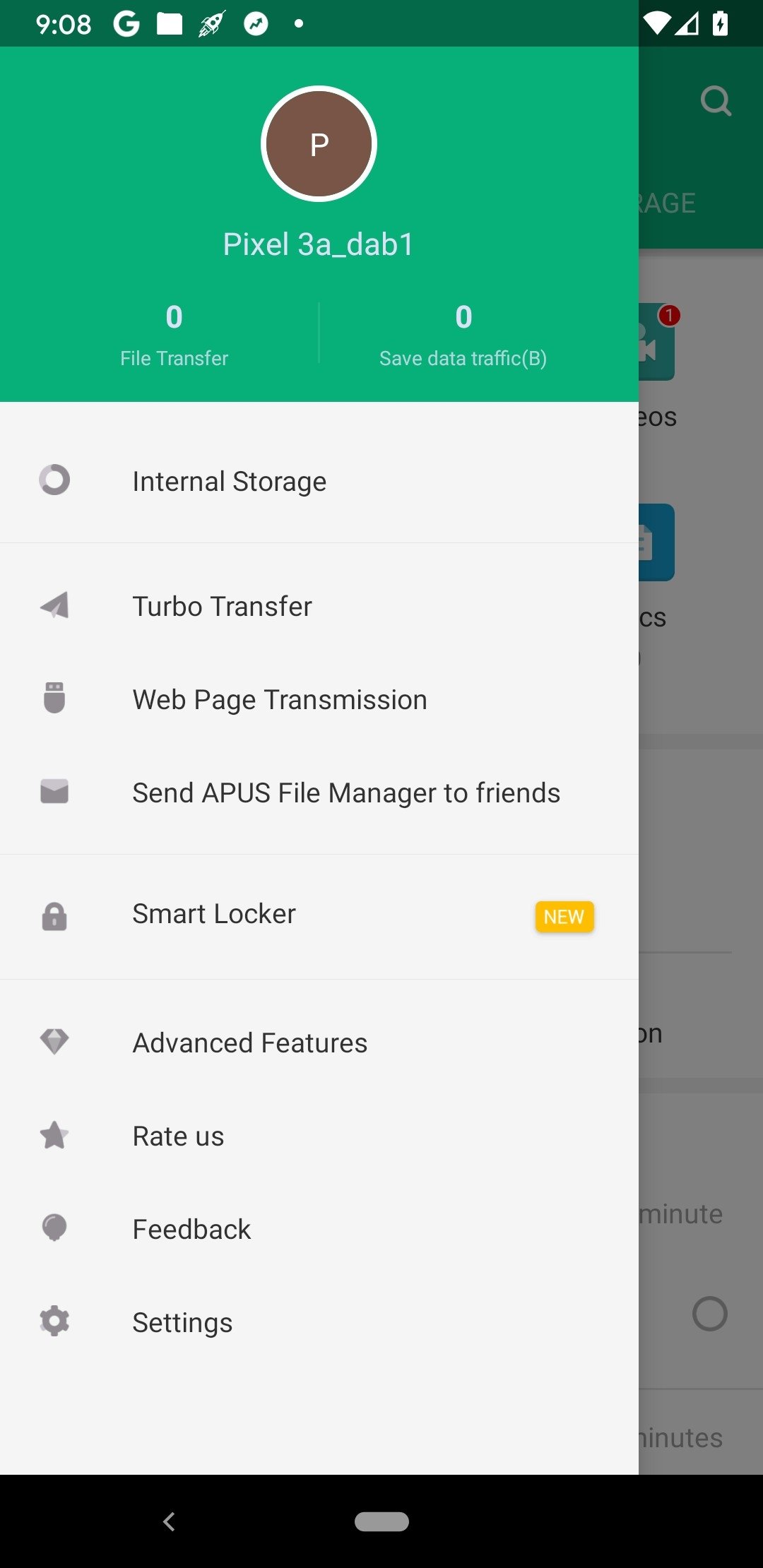The image displays a screenshot of an iPhone app interface, structured into a distinctive layout with one-third of the screen occupied by a green section at the top and the remaining two-thirds by a white section. 

In the green top section, there is a circle centered with a small letter "P," followed by the text "Pixel 3A-DAB1." Below, the app displays two status indicators: "File Transfer: 0" on the left and "Save Data Traffic: 0" on the right. 

The bottom white section consists of various menu options arranged in a typical list format. Each menu item has an icon on the left side and its description on the right. The options listed are as follows:
1. Internal Storage
2. Turbo Transfer
3. Web Page Transmission
4. Send APUS File Manager to Friends
5. Smart Locker (notably, with a "New" label to its right)
6. Advanced Features
7. Rate Us
8. Feedback
9. Settings

The screenshot appears to be highlighting the "Smart Locker" feature, as indicated by the "New" icon beside it, suggesting it is a recently added or updated function within the app.